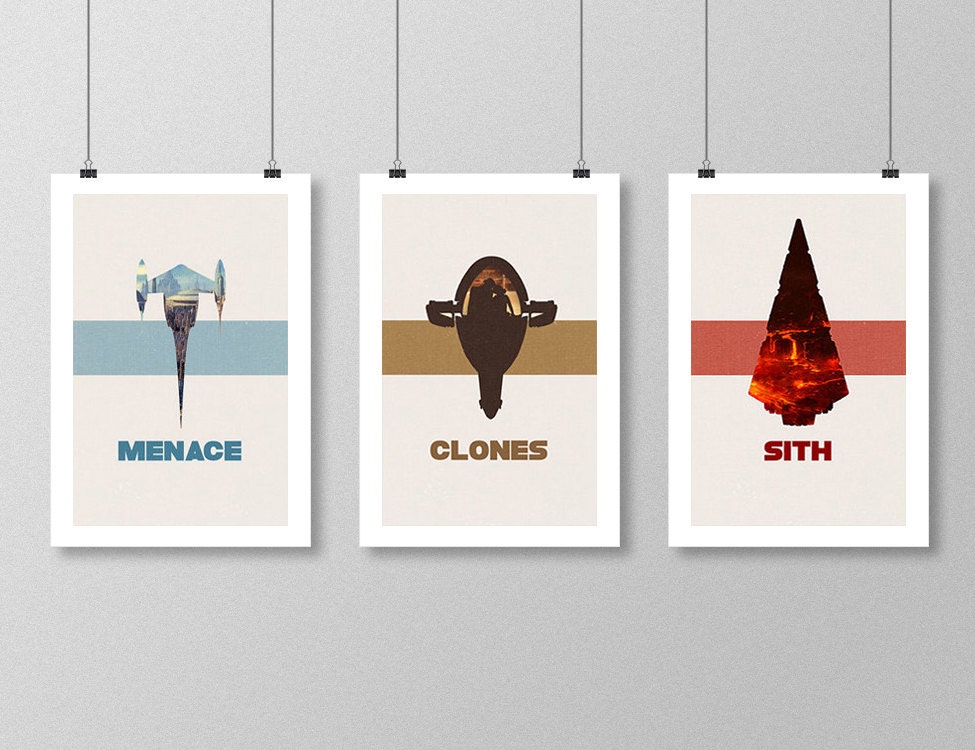This image depicts three parallel, vertical rectangular cards hanging against a gray wall. Each card is suspended by two thin black cords attached to the upper corners with small black clips. The cards are evenly spaced and aligned, with each featuring a narrow white border along the edges.

The left card showcases an image of a blue spacecraft above a horizontal light blue band that spans the center. Below the image, the word "menace" appears in uppercase blue text. The central card presents an illustration resembling a brown craft or helmet, positioned above a brown band that extends across the middle. At the bottom of this card, the word "clones" is displayed in brown font. The right card contains the depiction of a red and black spearhead or arrowhead-like shape set against a horizontal reddish band across the center. The word "Sith" is inscribed in red beneath the image.

All three cards follow a consistent design format, each with a central band matching the font color of the inscription below the respective image.